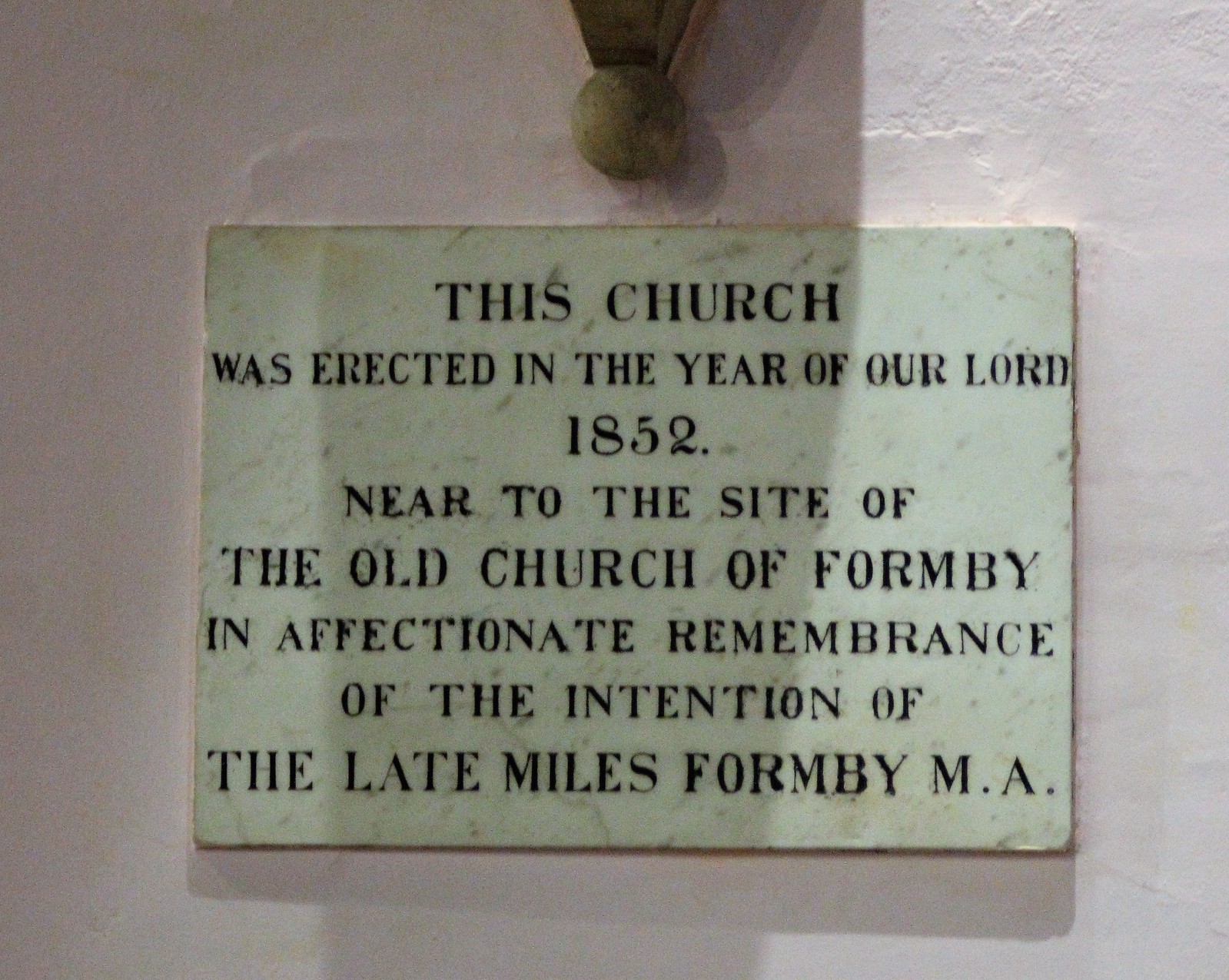The image depicts an aged plaque mounted on a textured, white-painted wall. Above the plaque, there is an ornamental fixture that resembles a triangular shape leading into a bowl, casting a shadow over the area. The plaque itself, more slate white in contrast to the brighter white of the wall, has a smooth yet well-worn appearance with a few roughened edges. The black text on the plaque, in an old-fashioned sans serif font, reads: "This church was erected in the year of our Lord, 1852. Near to the site of the old church of Formby, in affectionate remembrance of the intention of the late Miles Formby, M.A." The uneven layers of paint on the wall and the shadow cast by the fixture accentuate the historical ambiance of the site.